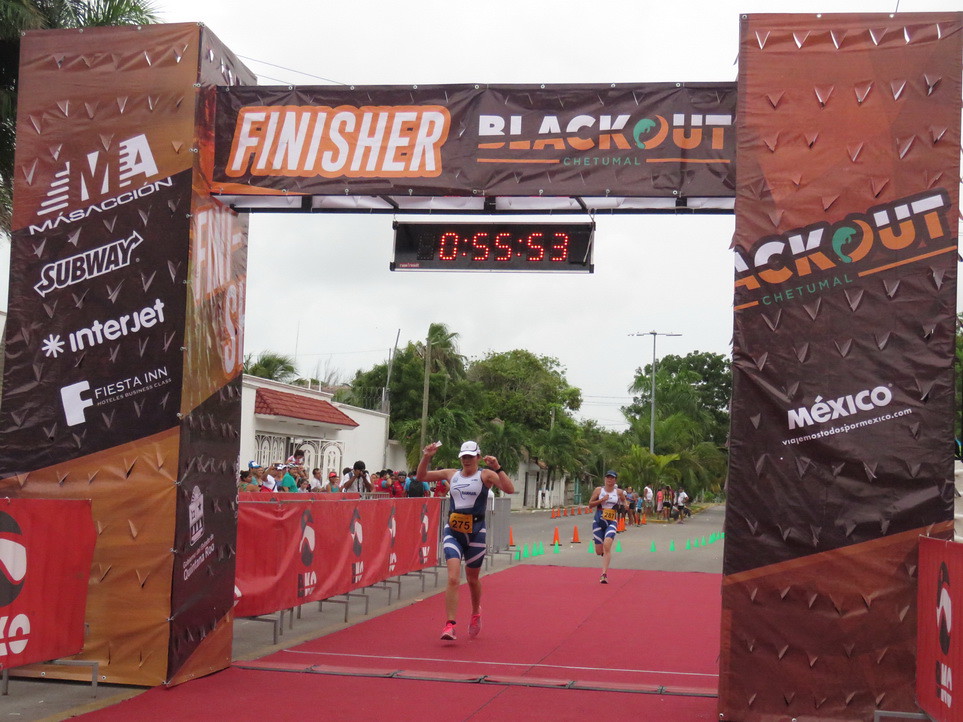This photograph captures the exhilarating moment at the finish line of a marathon, featuring a woman in a white tank top and blue-striped shorts with pink jogging shoes, triumphantly raising her hands as she is on the verge of crossing the line. The finish line comprises brownish blocks with a dark rectangle spanning across, emblazoned with the words "Finisher Blackout" in white. Above the finish line, a time clock displays an impressive finish time of 55 minutes and 53 seconds. A few feet behind her, another runner, whose gender is indistinguishable, can be seen hustling but dressed similarly in blue-striped shorts and a white top, just like the leading woman. Both runners appear determined as they stride on a red carpet towards the makeshift gate marking the race's conclusion.